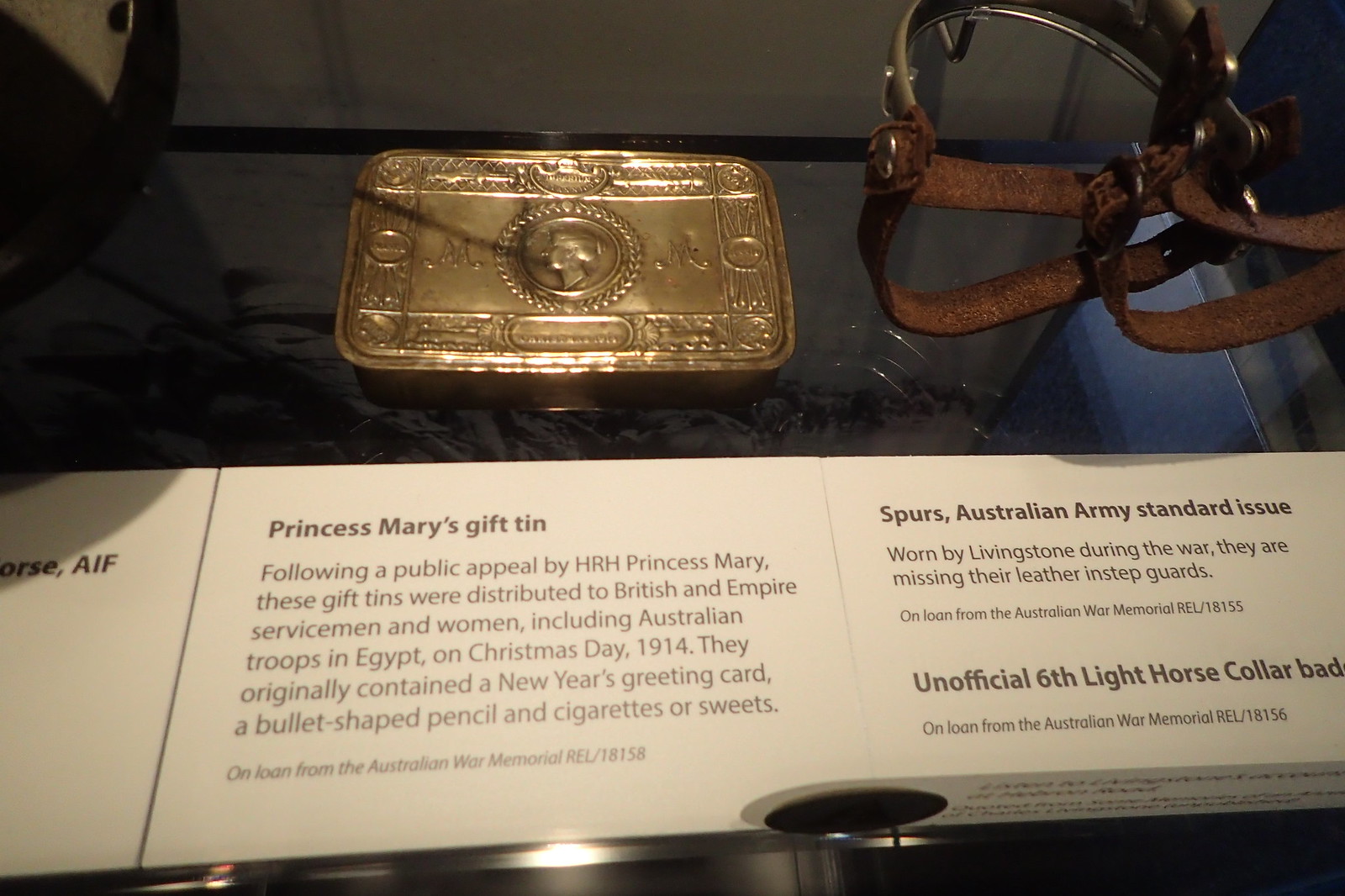The image depicts a museum display showcasing several historical artifacts lying on a glass table. Central to the display is a golden tin, labeled as "Princess Mary’s Gift Tin," with a detailed description. This tin was part of a charitable initiative by HRH Princess Mary, distributed to British Empire servicemen and women, including Australian troops in Egypt, on Christmas Day 1914. The original contents of the tin included a New Year's greeting card, a bullet-shaped pencil, and either cigarettes or sweets. In addition to the tin, on the right side, there is a set of horse spurs identified as Australian Army issue, with accompanying text that mentions they were worn by Livingston during the war. The display is set against a white background with black text descriptions, and other visible items include a buckle and a strap. The colors in the image range from gold and silver to brown, black, and various shades of white and gray, suggesting a carefully curated museum exhibit indoors.